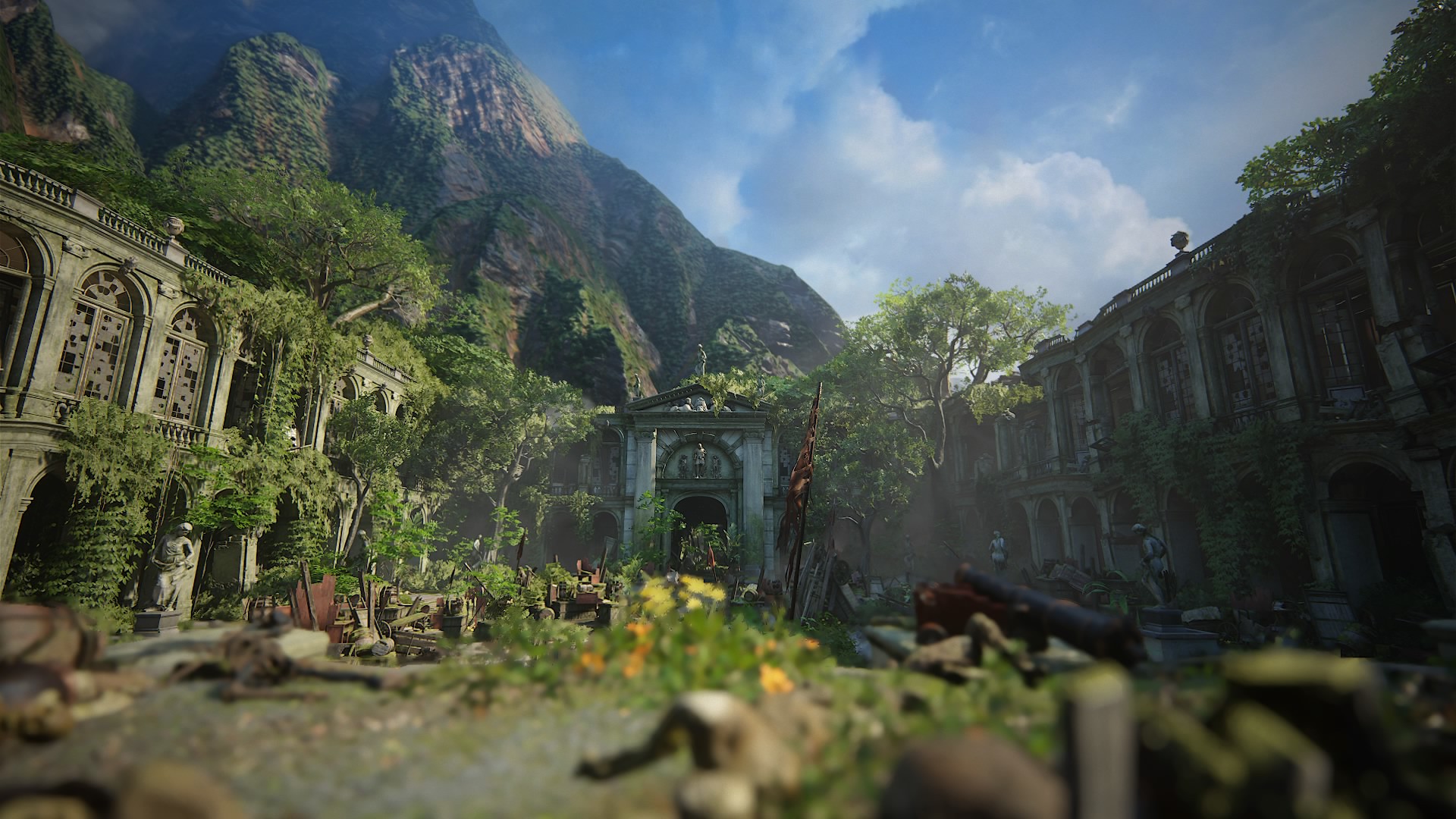In this captivating outdoor scene, ancient ruins stretch across a valley nestled below a towering, rocky mountain that ascends majestically into a clear blue sky dotted with fluffy white clouds. The rugged mountain's steep slopes dominate the right side of the image, while its base touches the middle, partially obscuring the remnants of old stone buildings. The blurred foreground reveals scattered rocks interspersed with vibrant yellow and orange wildflowers amidst lush green foliage. Trees, their branches weaving through the decaying structures, add a touch of nature's resilience to the historical tableau.

The ruins, constructed from a light, concrete-colored stone, feature numerous arched windows and intricate carvings atop each building, showcasing the architectural marvels of a bygone era. Central to the scene, an imposing stone entryway with columns flanking an arched opening stands prominently, crowned by a diamond-shaped detail above the doorway. Rows of windows, repeatedly adorned with arches, line the sides of the dilapidated structures, suggesting former grandeur.

Amongst the ruins, two figures can be seen towards the right-hand side. Dressed in white shirts, one individual is distinguishable by his white hat. Both appear engrossed in exploring the historical wreckage, adding a human element to the serene yet poignant atmosphere of historical decay reclaimed by nature.